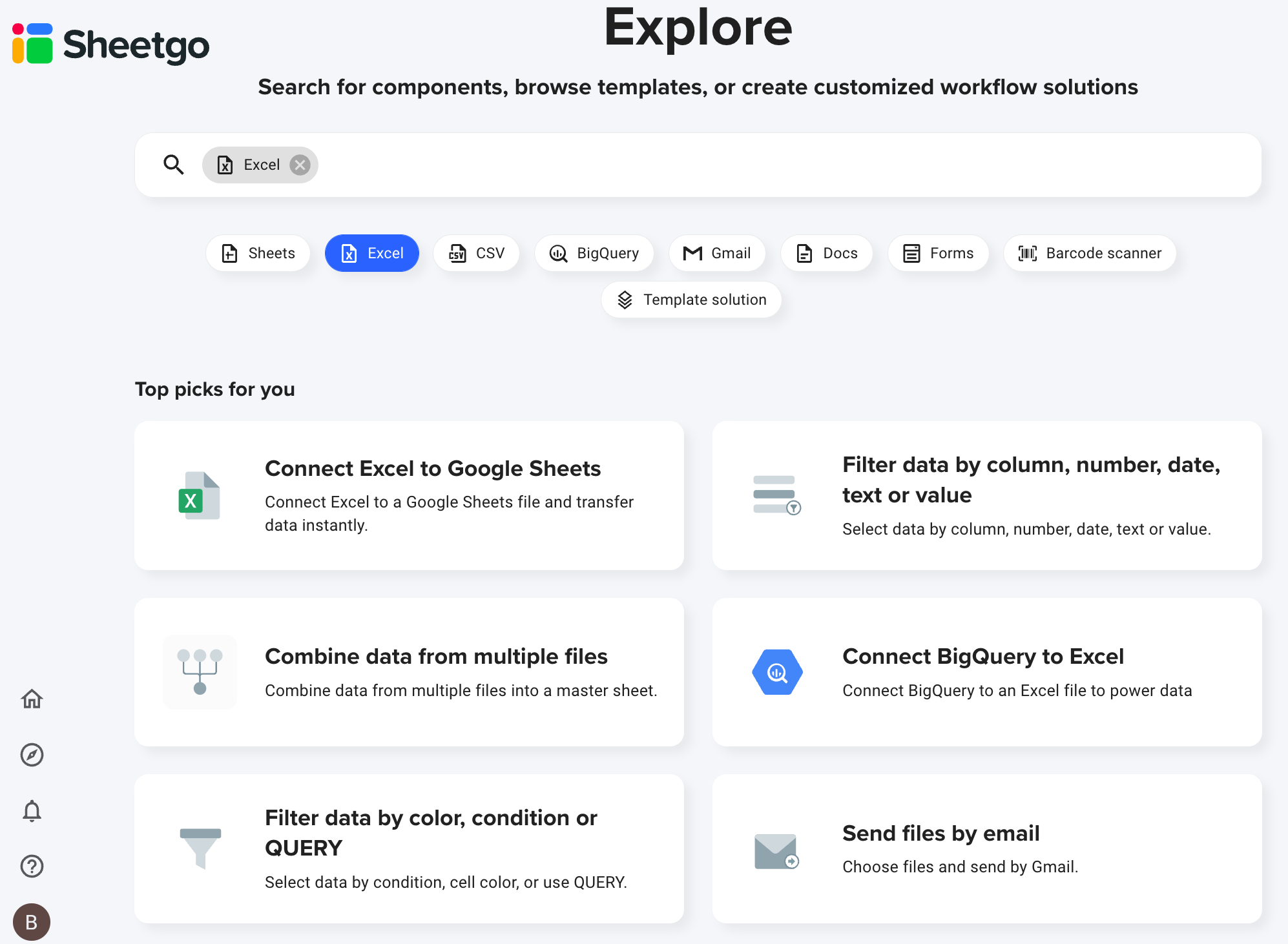The vertical-image displays a digital interface that you might encounter on a computer or smartphone device with a predominantly gray background. In the upper left-hand corner, the text "Chico" is prominently featured in black font, accompanied by a red circle, a green square, an orange cylinder, and a blue cylinder as part of its iconography.

Centered more significantly on the image is the bold black word "Explore." Beneath this, in a smaller font, the text reads: "Search for components, browse templates, or create customized workflow solutions." Directly below this description is a white search bar featuring a magnifying glass icon. The word "Excel" is written inside the bar, with an 'X' icon present to clear the search term.

Under the search bar are clickable options, including: Sheets, Excel (highlighted in blue), CSV, BigQuery, Gmail, Docs, Forms, Barcode Scanner, and Template Solution, each accompanied by a small icon. 

The section marked "Top Picks for You" is bolded in black, followed by six white, rounded rectangular boxes featuring text and an icon. They read as follows:
1. Connect Excel to Google Sheets
2. Combine data from multiple files
3. Filter data by color, condition, or query
4. Filter data by column, number, date, text, or value
5. Connect BigQuery to Excel
6. Send files by email

At the bottom left-hand side of the interface, there are several icons, including a home, a circle with lines, a bell, a question mark, and a filled circle with a white 'B.'